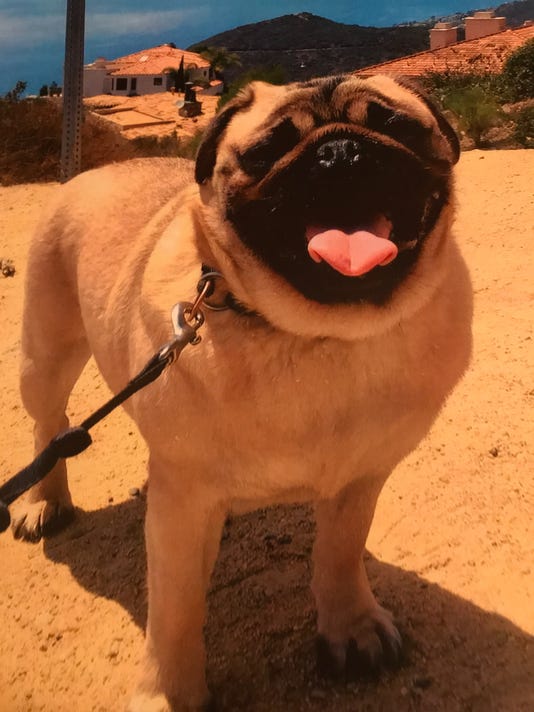The image features a small dog, likely a pug, with a distinct wrinkled, scrunched-up face, characterized by a black nose, black ears, and dark fur around its eyes and mouth. Its tongue is hanging out, revealing a happy expression. The dog has a light tan coat and short legs, standing on a light brown dirt surface that suggests a dry, possibly desert-like area. The dog is facing the camera, casting a shadow in the direct sunlight. A black leash with a silver clip is attached to its collar on the left side. In the background, there are green trees, bushes, and vegetation covering a hillside, along with rooftops of houses with red clay tiles. A silver signpost is also visible. The sky is blue with some white clouds, indicating it's daytime.